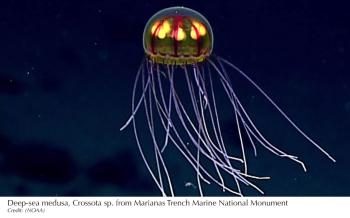The image depicts a deep-sea medusa, specifically a Crossota species, from the Mariana Trench Marine National Monument. The creature, resembling a jellyfish, features a dome-like head adorned with cranberry-red veining and what appears to be three yellow, heart-shaped structures that are illuminated, suggesting bioluminescence. Long, fibrous tentacles extend from the base, creating a striking visual contrast against the dark, murky underwater background. Despite its otherworldly appearance that evokes the look of a delicate, glowing sculpture or lampshade, the detailed caption confirms its authenticity as a real-life deep-sea inhabitant. This photograph, small and rectangular, captures the extraordinary and somewhat ethereal beauty of the deep-sea medusa, emphasizing its unique adaptations to one of the most extreme environments on Earth.